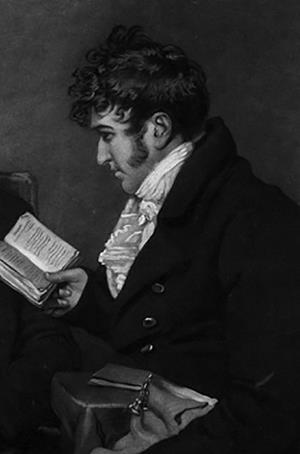The image depicts a black-and-white drawing or painting of a man in profile view, seated and reading from a small book held chest-high in his right hand. His hair is dark, shaggy, and somewhat unruly, accentuated by prominent, long sideburns. He wears an old-fashioned outfit consisting of a dark, long-sleeved, button-down jacket and a poofy white shirt with a high collar peeking out in front. The man's pants are light-colored, providing a slight contrast to the primarily dark composition. The background appears charcoal-y, contributing to the overall somber, monochromatic tone of the scene. Despite the comic-like, unrealistic elements of the drawing, the detailed portrayal of the man suggests a period setting, possibly from the 1800s. There is no text or other colors in the image, just shades of black and white.